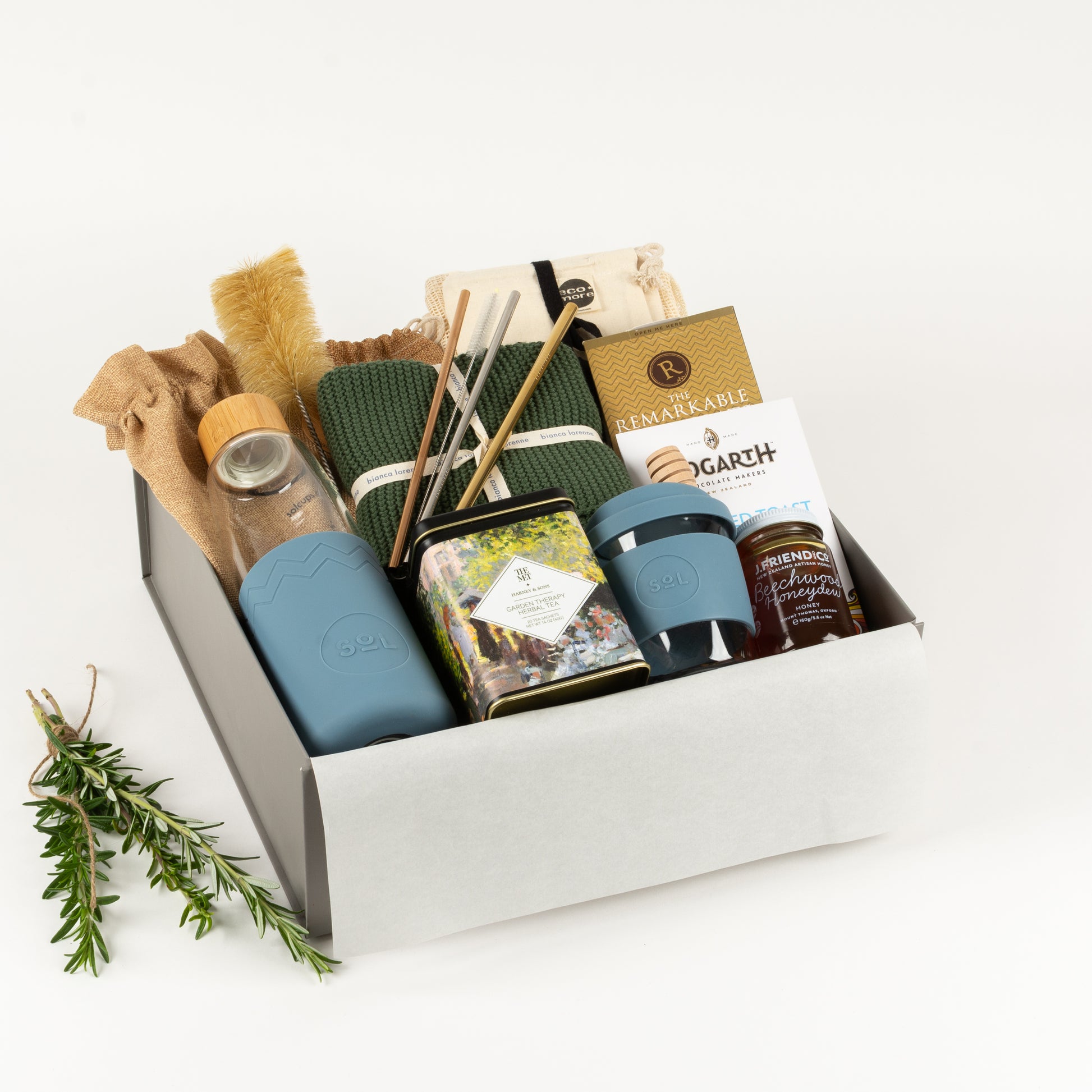The image is a meticulously staged, full-color photograph of a rectangular, shoebox-sized, gray cardboard gift box set against a gradient light gray to near white background. The box is positioned at an angle, with the open lid revealing an assortment of carefully arranged items. Notable contents include a small brown wire brush, a clear glass bottle with an orange lid and an insulated blue base, green socks or a green sweater, a brown burlap sack, and a couple of unspecified container items with tiny print on them. Additionally, there is a tin can, possibly of tea, and a smaller jar labeled "GARCH." The items are placed in a bed of tissue paper, and to the lower-left corner of the box, a bundle of green stem-like plants, tied with string, adds a touch of natural, woodland-themed aesthetics. The colors in the box range from light blue, dark green, tan, light brown, to black, creating a warm, nature-inspired palette. The photograph is taken from a slightly elevated side angle, looking down at the contents.